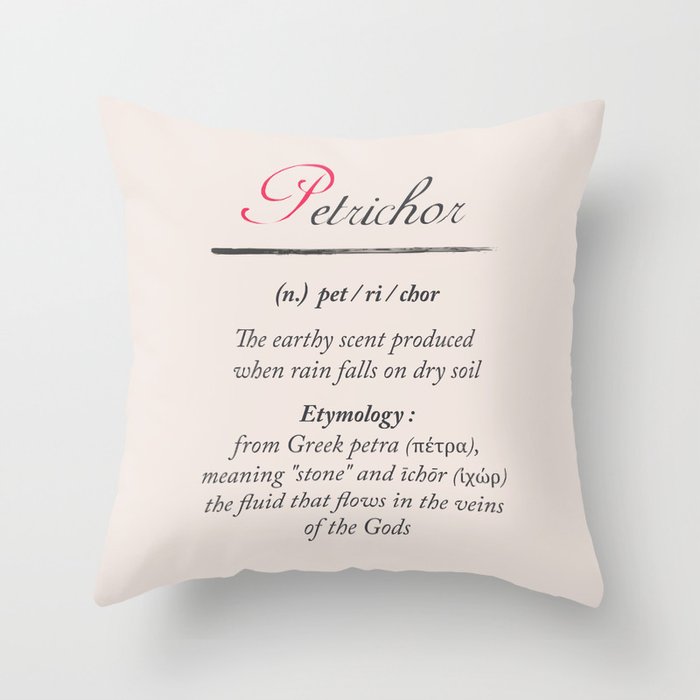This image features a square, white throw pillow with a detailed inscription on it, positioned centrally against a blank, white background. The pillow is described as fluffy and has a slightly contoured shape with pointed ends. At the top of the pillow, the word "Petrichor" is written in cursive, with the "P" highlighted in red and the rest of the letters in black. Below "Petrichor," there is an underline, followed by a dictionary-like definition in italics that reads, "the earthy scent produced when rain falls on dry soil." Further down, in bold, the word "Etymology" is displayed, followed by an explanation that says, "from Greek Petra, meaning stone, and Ichor, the fluid that flows in the veins of the gods." The text is arranged vertically from the top to the bottom of the pillow. The setting emphasizes the serene and minimalistic presentation of the pillow with its poetic and scholarly text.